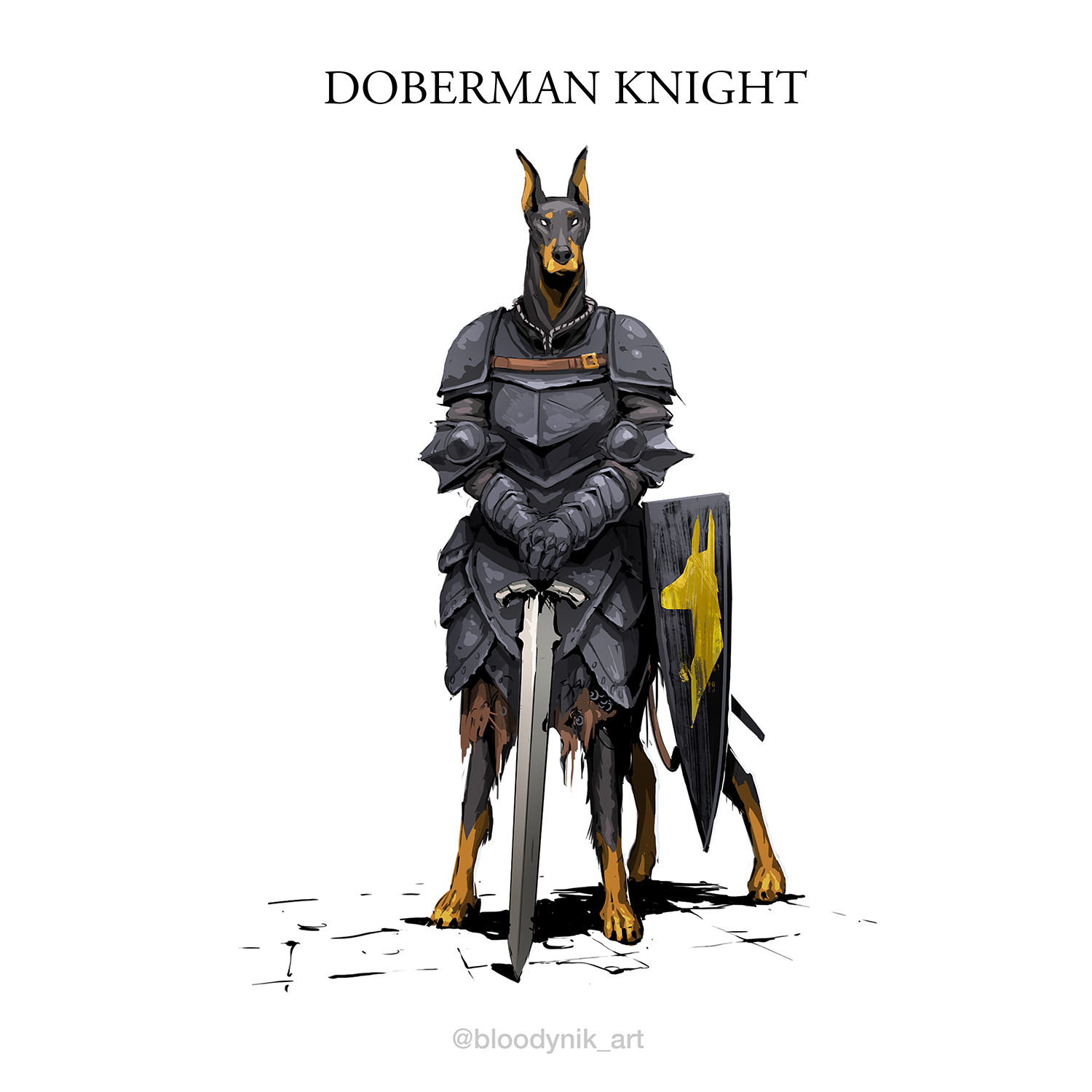The artwork depicts a Doberman knight in a centaur-like form, standing tall on a white brick-tiled path. The Doberman, with its distinct black and tan coloring, is clad in an elaborate suit of knight's armor. The armor is predominantly silver with a brown strap across the chest, resembling a belt, and has hints of red or brown cloth peeking underneath. The Doberman's front legs blend into a human-like upper body, with its head emerging from the top of the armor. Its paws are crossed over a silver sword that it holds with a serene yet imposing presence. To its right, a black shield featuring a yellow dog emblem leans against its armored body. Behind it, a glimpse of the Doberman’s tail is visible. The entire scene is set against a white background, with the text "Doberman Knight" in black at the top. At the bottom, the artist’s signature "[@bloody.nick_art](https://www.instagram.com/bloody.nick_art)" is noted, emphasizing that this is likely a digital painting or drawing. The overall effect is both majestic and otherworldly, as the knightly Doberman commands attention with its noble stance and detailed attire.